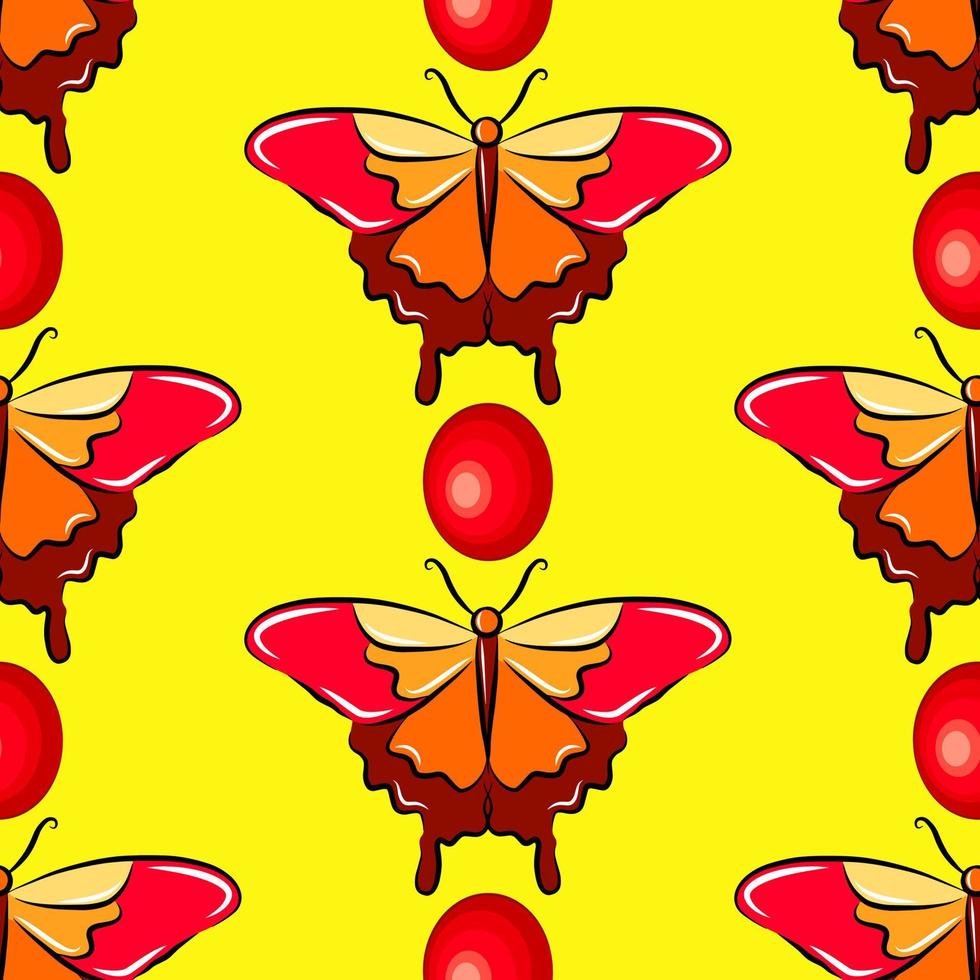This highly stylized digital artwork features a repeating pattern of brightly colored, butterfly-like insects set against a vivid yellow background. The butterflies, rendered in shades of red, brown, yellow, and touches of orange, create a mirrored effect with two full butterflies in the center and partial wings on either side, implying the continuation of the pattern beyond the frame. Between each butterfly, both vertically and horizontally, are distinct, egg-shaped objects that are primarily red but fade to lighter red and white towards their centers. The butterflies appear as if they are melting, adding a glossy and almost surreal quality to the image.